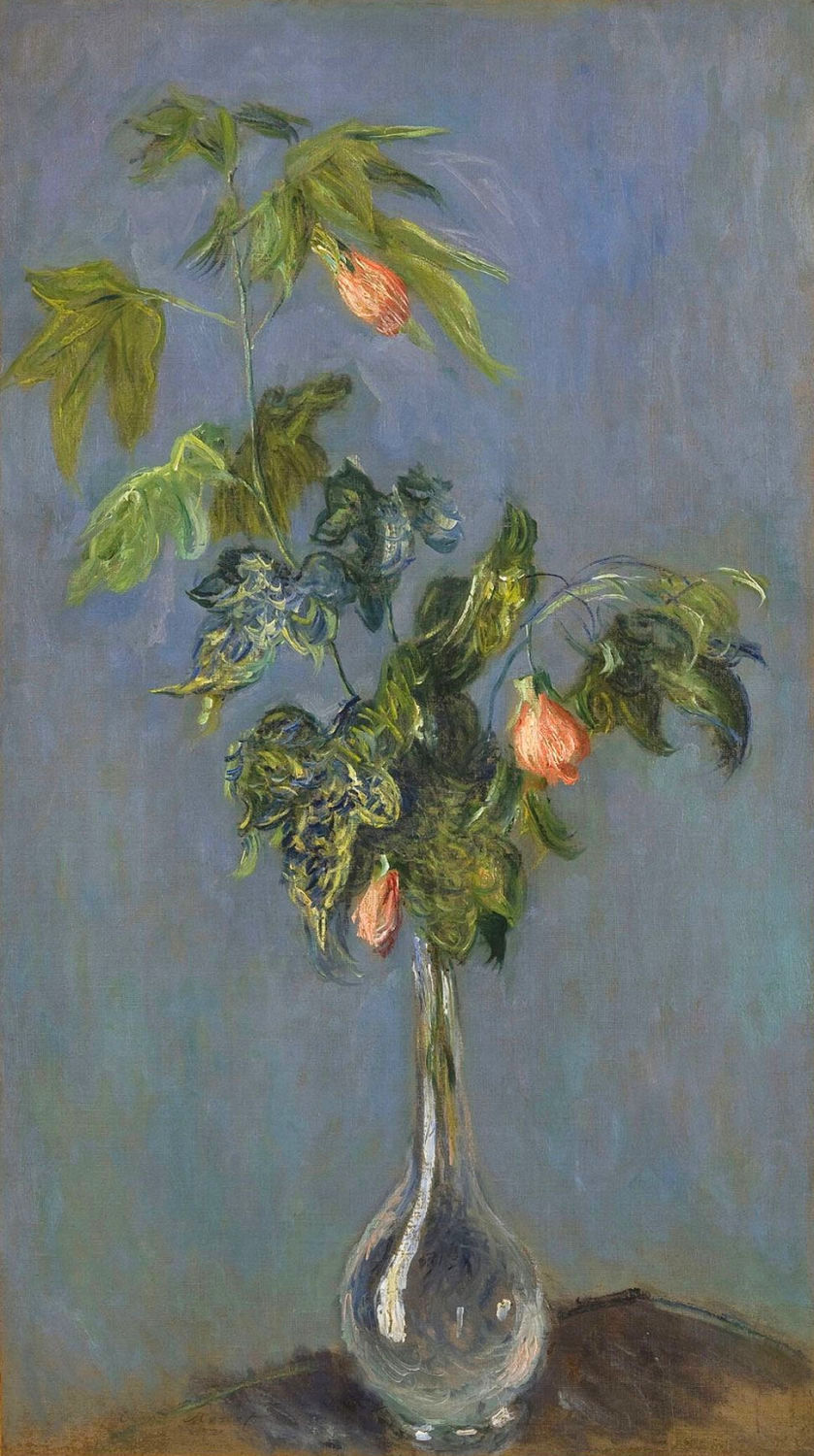This detailed oil painting presents a captivating still life composition of a clear, thin-stemmed glass vase filled with water, sitting elegantly on a dark brown wooden table. Emerging from the vase are three distinctive orange blossoms, subtly poised downwards, signifying perhaps either their opening or dying stage. These flowers are accompanied by about three to four green branches that vary in shade, with some leaves appearing dark green while the upper section boasts lighter hues. The vase's transparency allows a glimpse of both the blue back wall and the green stems within. The backdrop is an intriguing blend of purple, green, and possibly light blue splotches, adding an abstract quality to the otherwise simple and elegant setting. The thoughtful use of light from the left further accentuates the delicate details of the blossoms and leaves, creating a beautiful contrast against the rich tones of the table and the vibrant background.